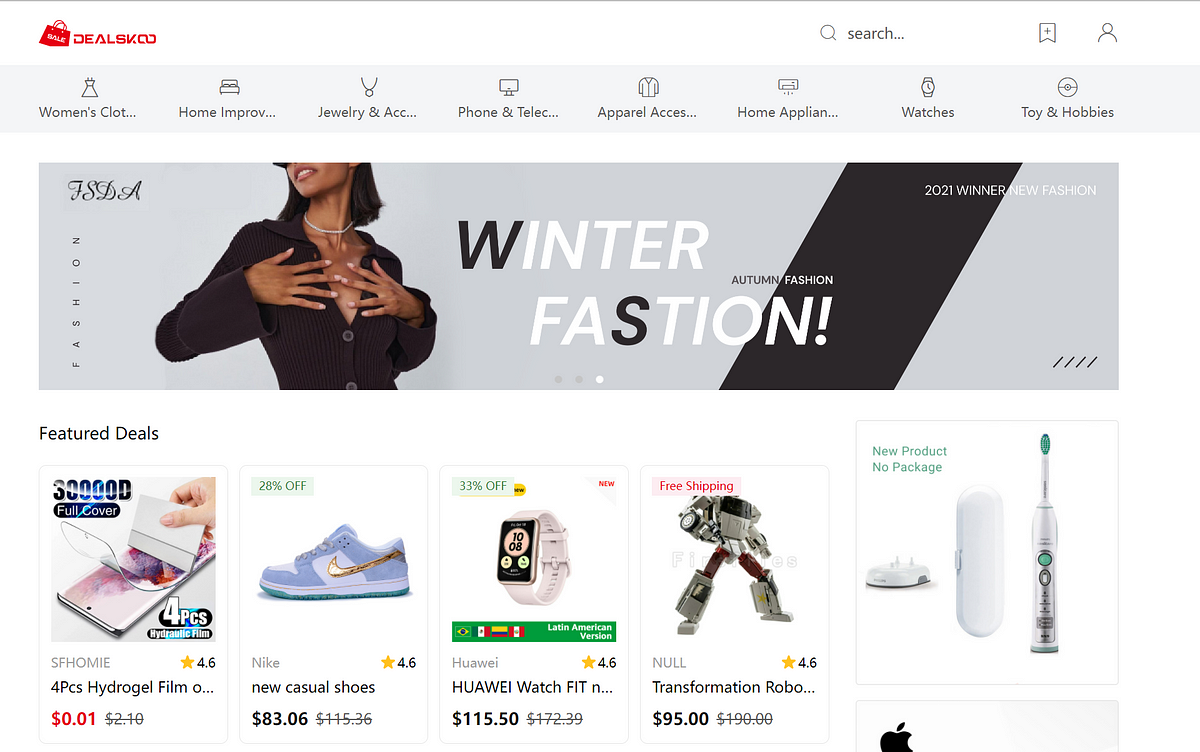**Detailed Screenshot Description:**

The screenshot is from a webpage with the header displaying "dealsk.co" in bold red lettering on the top left. On the top right, there is a search icon represented by a magnifying glass, next to a square icon with a plus symbol and a silhouette of a person.

Below the header, there are several categories with corresponding icons:
- **Women's Clothing**: Represented by an illustration of a dress.
- **Home Improvement**: Illustrated by a bed icon.
- **Jewelry and Accessories**: Shown by an icon of a necklace.
- **Phones and Telecommunications**: Depicted by a TV icon.
- **Apparel Accessories**: Represented by a shirt icon.
- **Home Appliances**: Illustrated with what appears to be an oven.
- **Watches**: Shown by an icon of a wristwatch.
- **Toys and Hobbies**: Represented by a Pokémon ball.

Moving further down, an image under the "Fashion" section shows a woman wearing a black dress. Her dress is provocatively styled, with her hands on her breasts, partially exposing them. She is adorned with a white necklace. Above her image, there are additional descriptors: "Winter Fastion" (noting the misspelling of 'fashion'), "Autumn Fashion," and "2021 Winter New Fashion."

Below this section, there is a display of featured deals:
- **Four Piece Hydrogel Film**: Shows a phone with a cover, priced at $0.01.
- **New Casual Shoes**: Priced at $83, marked as 28% off, showing a pair of white shoes with a gold checkmark on them.
- **Hawaii Watch Fit**: A smartwatch priced at $115, with a 33% discount.
- **Free Shipping Transformation Robot**: Displayed as a gray robot, priced at $95.
- **New Product - No Package**: Shows a white electric toothbrush alongside a white box.